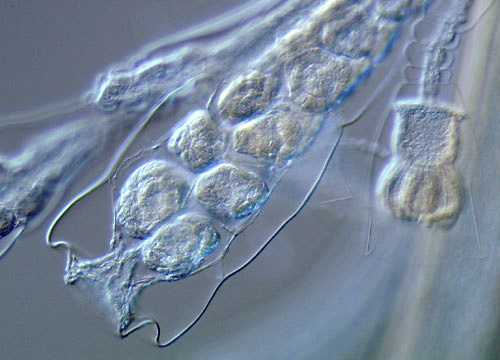This image is a highly detailed microscopic view showing a complex translucent film with a prominent blue and white color scheme. The background primarily consists of swirling blue hues layered over a gray backdrop. The microstructure is characterized by white raised bumps and intricate textures that create a pebble-like appearance. Notably, there's a distinctive section starting from the center and extending towards the bottom left, resembling a tail or a transparent worm with a wire outline. This section features gelatinous, block-like formations along its length and includes a rounded tip reminiscent of a gloved fist. The right side of the image presents another similar structure with a wide, bulbous head and a thick central line, enhancing the impression of a segmented, jellyfish-like entity under magnification.